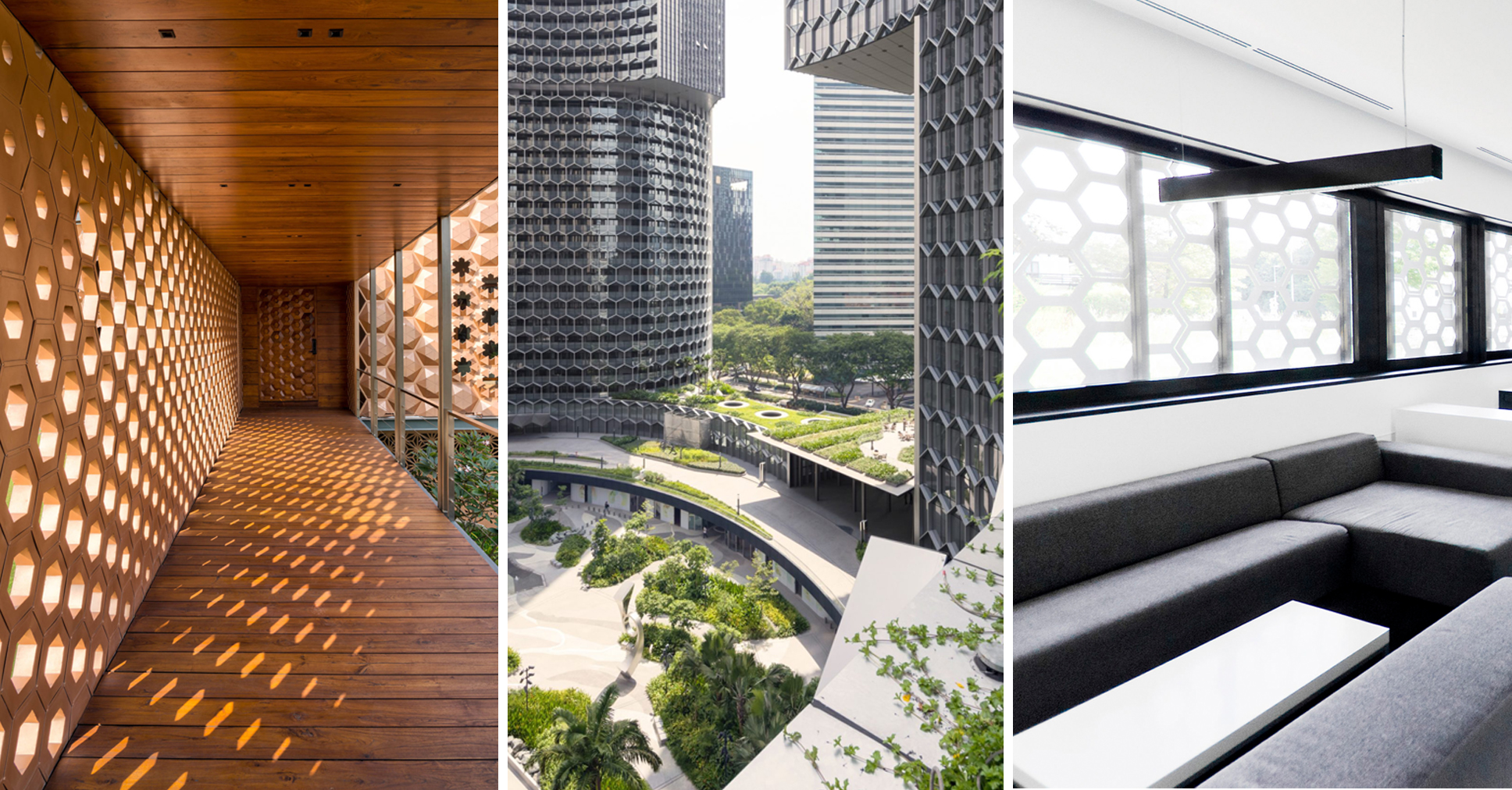The image consists of three aligned, vertically rectangular photographs placed side by side. The left photograph showcases a wooden walkway leading to a planked wooden patio, bordered by a banister on the right, which overlooks a garden below filled with trees. Sunlight filters through hexagonal-shaped cutouts in the wooden walls on the left, casting light patterns onto the walkway.

The center photograph features a cluster of high-rise buildings, possibly modern skyscrapers, that are partially silver with green areas and grass visible at their bases. The architectural design includes prominent hexagonal patterns, particularly noticeable in a building sign located at the top right corner, and a rounded high-rise on the left side.

The right photograph, presented in black and white, depicts an elegantly designed waiting area. The room is furnished with light gray sofas arranged in a rectangular layout around a white rectangular table in the center. The walls feature windows with an intricate hexagonal honeycomb pattern overlay, and a rectangular light fixture hangs from the ceiling, casting a sleek, modern ambiance to the room.